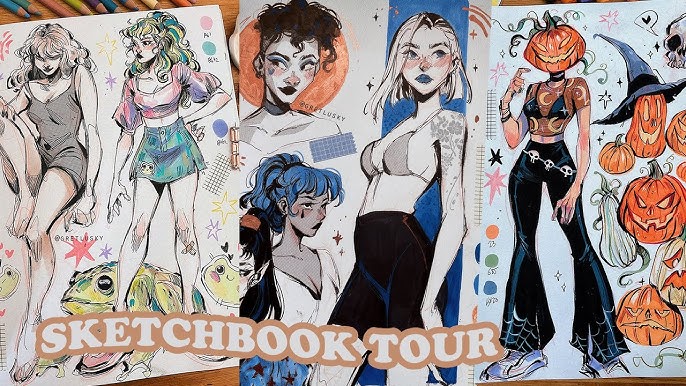This is an intricate spread from a sketchbook program by Gretel Lusky, showcasing a vivid array of characters. At the bottom, the image is labeled "Sketchbook Tour" in white lettering outlined in brown. On the left side, a detailed black-and-white sketch features a woman in a gray one-piece bathing suit standing atop a frog. Adjacent to her is the same character rendered in vibrant colors, sporting a turquoise and yellow hairstyle, a pink crop top, and a short turquoise skirt. Moving to the center, we observe multiple sketches: a woman with dark hair, heavy makeup, and an orange moon backdrop; below her, another character with blue hair in a messy ponytail and teardrop face paint; and a prominent figure clad in a gray bralette and black pedal pusher shorts, revealing a tattoo on her arm. The scene is completed with a right-side illustration of a character wearing a pumpkin mask atop her head, transparent shirt adorned with moons and stars over a black bralette, and black flared pants decorated with cobwebs. Alongside her, several jack-o'-lantern sketches, including one adorned with a witch's hat, add to the Halloween theme. The spread is detailed and colorful, capturing Lusky's diverse creative expressions.